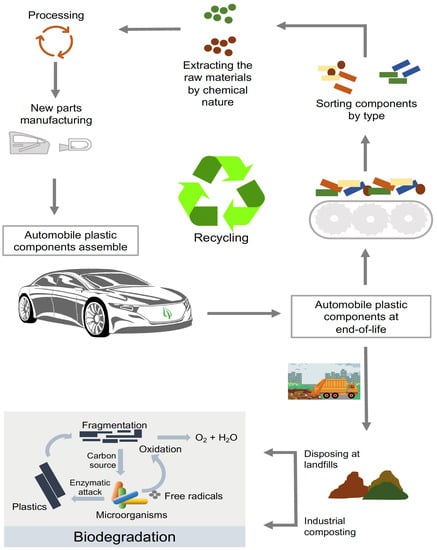The image depicts the extensive lifecycle of automobile plastic components, delineating the process from assembly to end-of-life recycling. Central to the diagram is a green recycling symbol accompanied by the word "recycling." This intricate flowchart illustrates two distinct pathways: one for biodegradation and another for recycling into new components. The biodegradation pathway, positioned below an image of a car, details the processes of fragmentation, carbon sourcing, and oxidation from free radicals, leading to disposal in landfills and industrial composting. The recycling pathway begins with the sorting of components by type, depicted by colored blocks transitioning into dots, and labeled as "extracting raw materials by chemical nature." Subsequent steps include processing (illustrated by circular arrows), new parts manufacturing (highlighted by drawings of car parts such as a door), and assembly of automobile plastic components into a vehicle. The cycle culminates in the depiction of the end-of-life stage, where these components re-enter the recycling process, creating a loop. The flowchart's arrows, gray in color and forming a figure-nine pattern, guide the viewer through each step, accentuated by vibrant colors such as red, blue, and green, providing a comprehensive overview of the automotive recycling process.